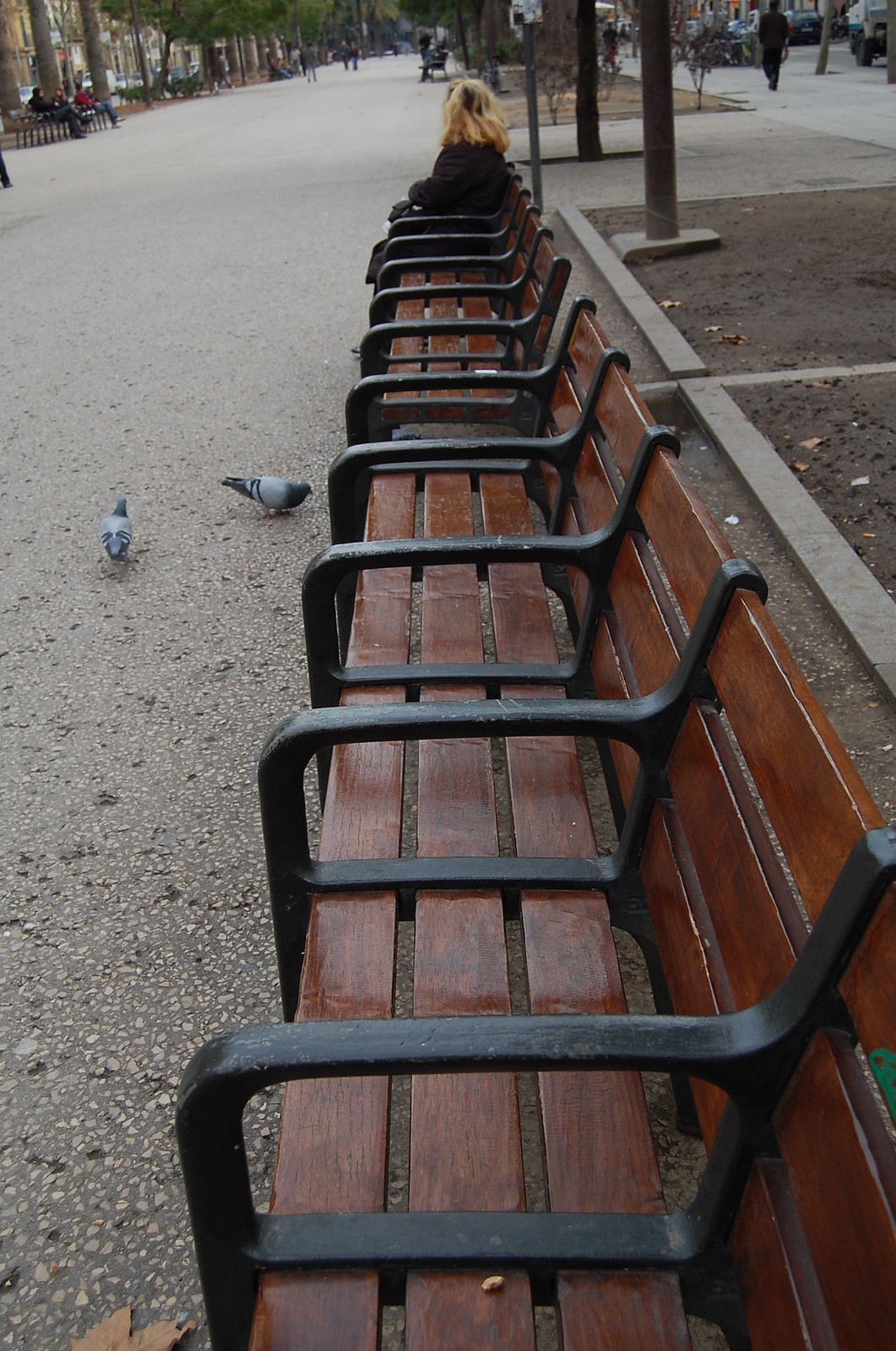This detailed color photograph captures a pedestrianized city walkway, adorned with a series of connected, dark brown-stained wooden park benches framed by black wrought iron armrests and railings. The viewpoint is from the end of this long row of benches, emphasizing their length and continuity. The walkway is pebble-paved, leading into the distance through what appears to be a city park area. Positioned at the far end of the benches is a woman with blonde hair and dark roots, dressed in black, sitting with her back slightly turned towards the viewer. Scattered pigeons peck at the ground in front of the benches, adding life to the tranquil scene. Flanking the benches are garden planters, possibly barren due to winter, and the bases of what seem to be street lamps. Surrounding the parkway are trees and people strolling, contributing to the lively yet serene atmosphere, reminiscent of an urban oasis, possibly akin to New York City.